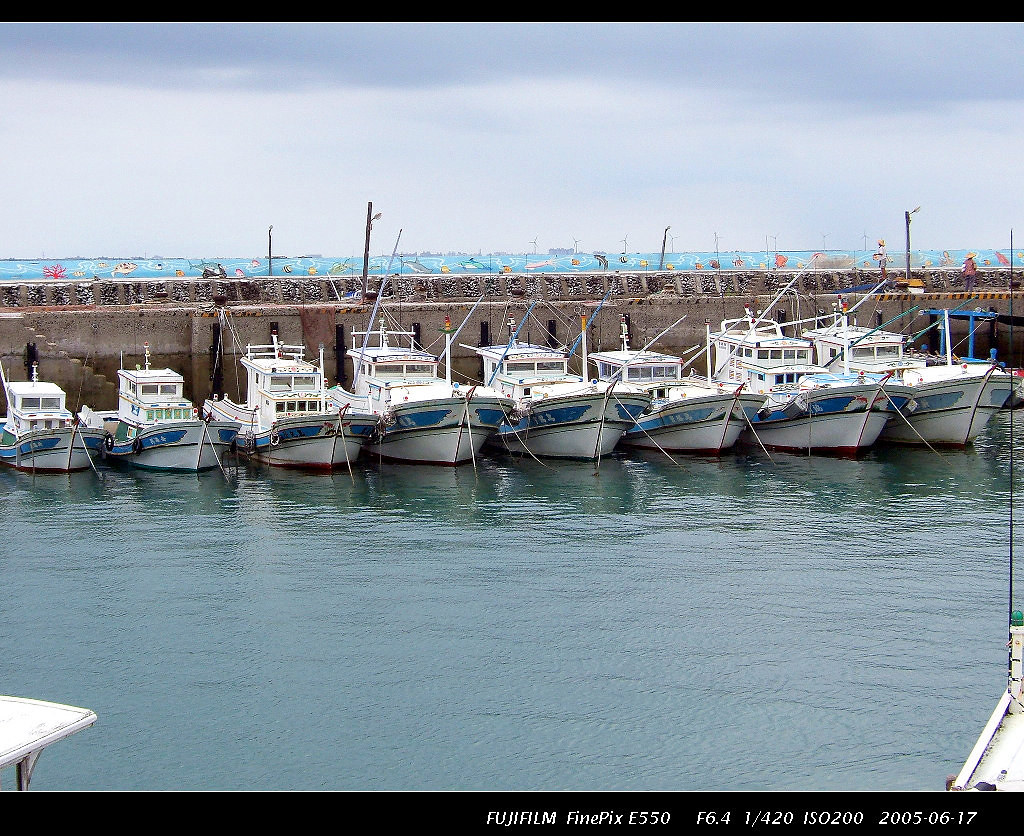This photograph, taken on June 17, 2005, with a Fujifilm FinePix E550 camera (settings: F6.4, 1-420, ISO 200), captures a serene marina scene. Eight white boats, each adorned with a distinctive blue stripe running along their edges, are lined up in a harbor, docked against a sturdy brown concrete wall. These boats, arranged in ascending order of size from left to right, feature small cabin areas and an overall similar design. The wall behind the boats includes steps leading down to the water level, poles likely intended for lights, and a colorful mural depicting ocean creatures. The sky in the background is partly cloudy, adding to the tranquil ambiance of the scene. At the very bottom of the image, technical details and the date are marked in white lettering against a black strip, reading "Fujifilm FinePix E550, F6.4, 1-420, ISO 200, 2005, 06, 17."